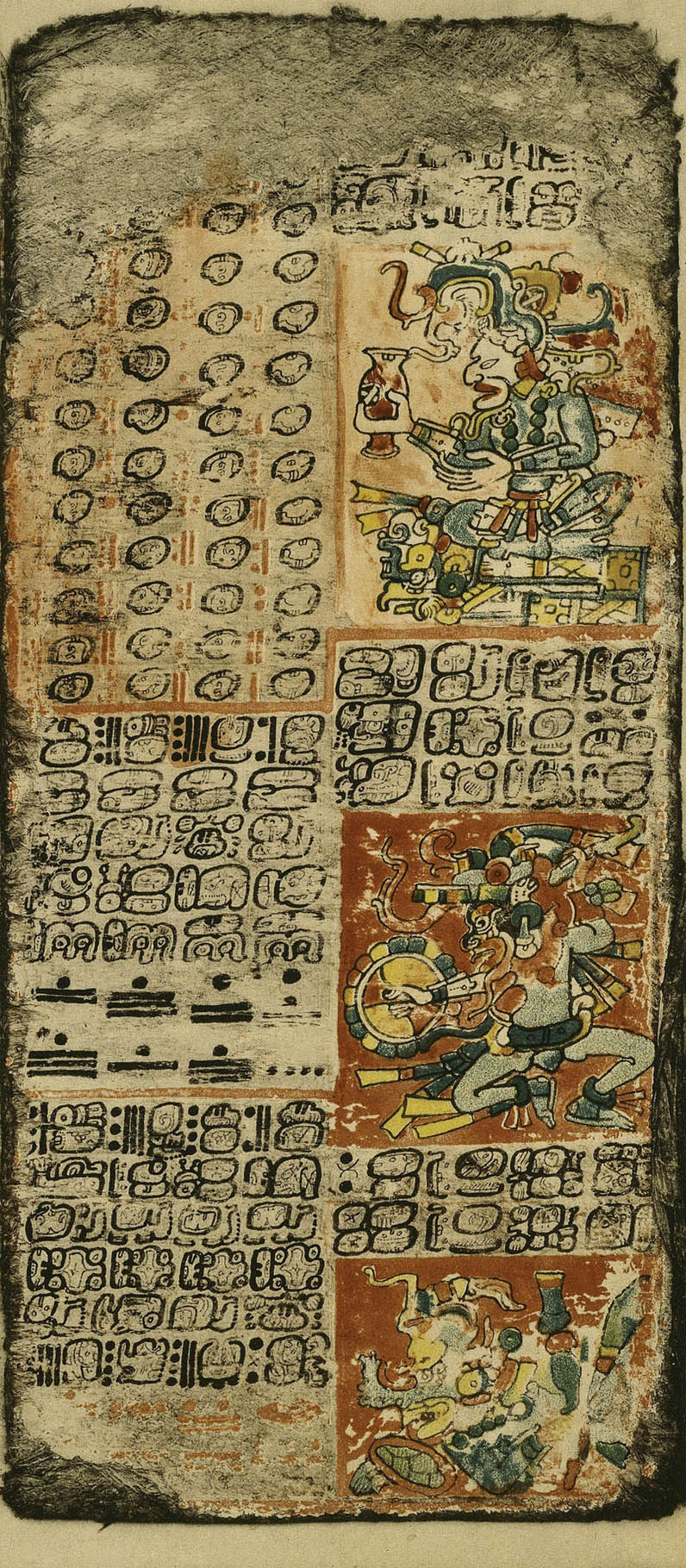The image depicts a detailed and worn Central or South American textile, likely of Aztec or Mayan origin. The textile is cream-colored and shows significant aging, with faded and rubbed-away sections, particularly at the top and the edges. Along the right side, there are vibrant, colorful panels showcasing a series of figures, possibly deities or kings. The top figure is adorned with an elaborate headdress and is depicted holding an object; colors like red, green, and blue still stand out. Below, another figure appears to be dancing with a red background, surrounded by intricate designs. The bottom figure looks human-like, also rich in colors such as yellow, orange, black, and green. Throughout the textile are additional smaller details and possible text in the native language, further emphasizing the rich cultural significance of this ancient artifact.